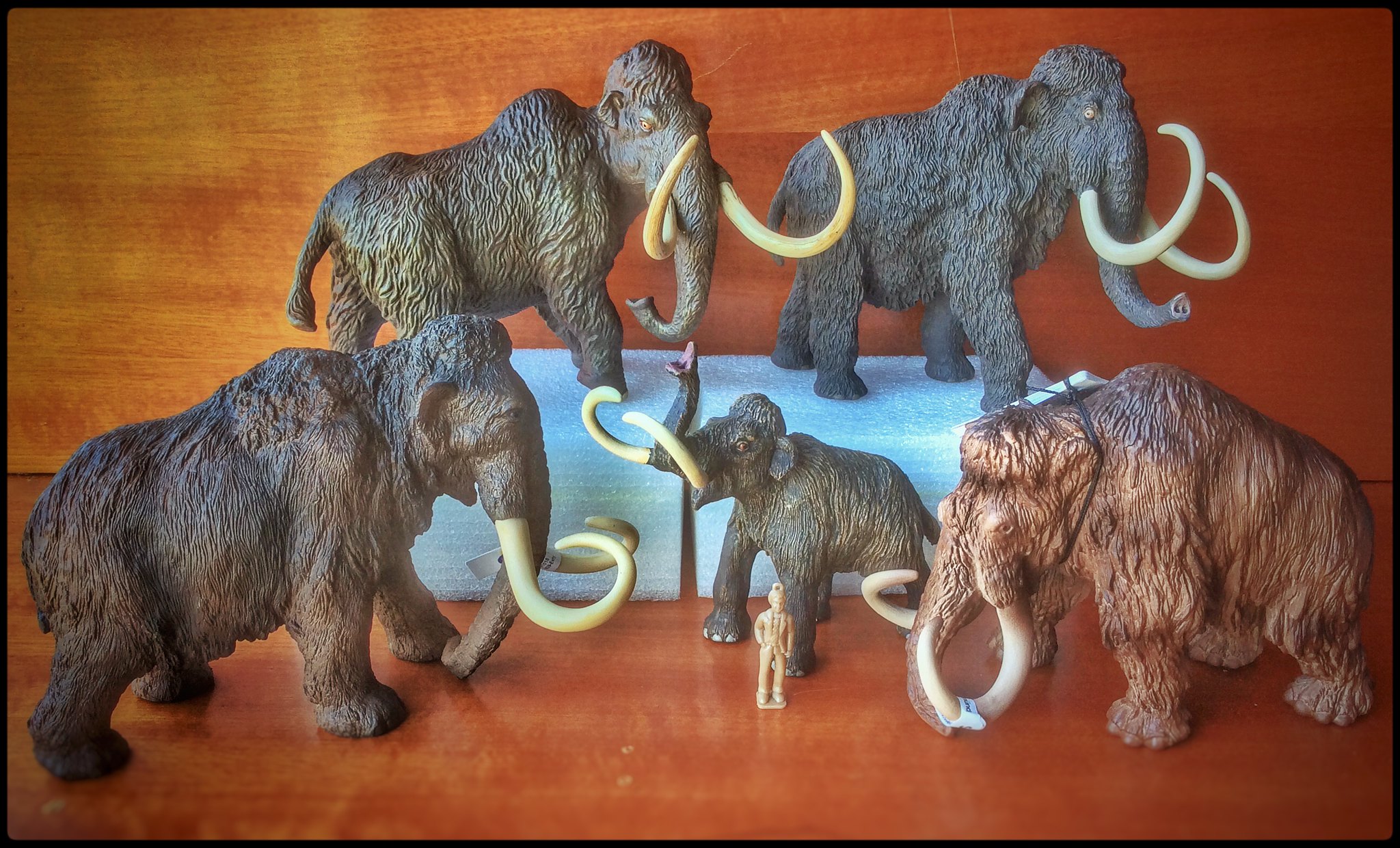The photograph features a group of five plastic woolly mammoth models displayed against a glossy brown wooden wall and table. Four of these mammoths are a charcoal gray color, while one is brown. Notably, the models have intricate details with long white tusks. Two of the gray mammoths are positioned on rectangular pieces of foam in the background, elevating their height and creating depth in the display. In the front row, on the outer edges, are two larger mammoths each adorned with a tag; the one on the left also has an elastic cord around its neck. The center of the front row showcases a smaller mammoth facing left. Additionally, a beige toy soldier figure stands between the mammoths, with its right hand in its pocket. The entire scene is captured indoors, and the reflections on the wood surface emphasize the glossy finish.